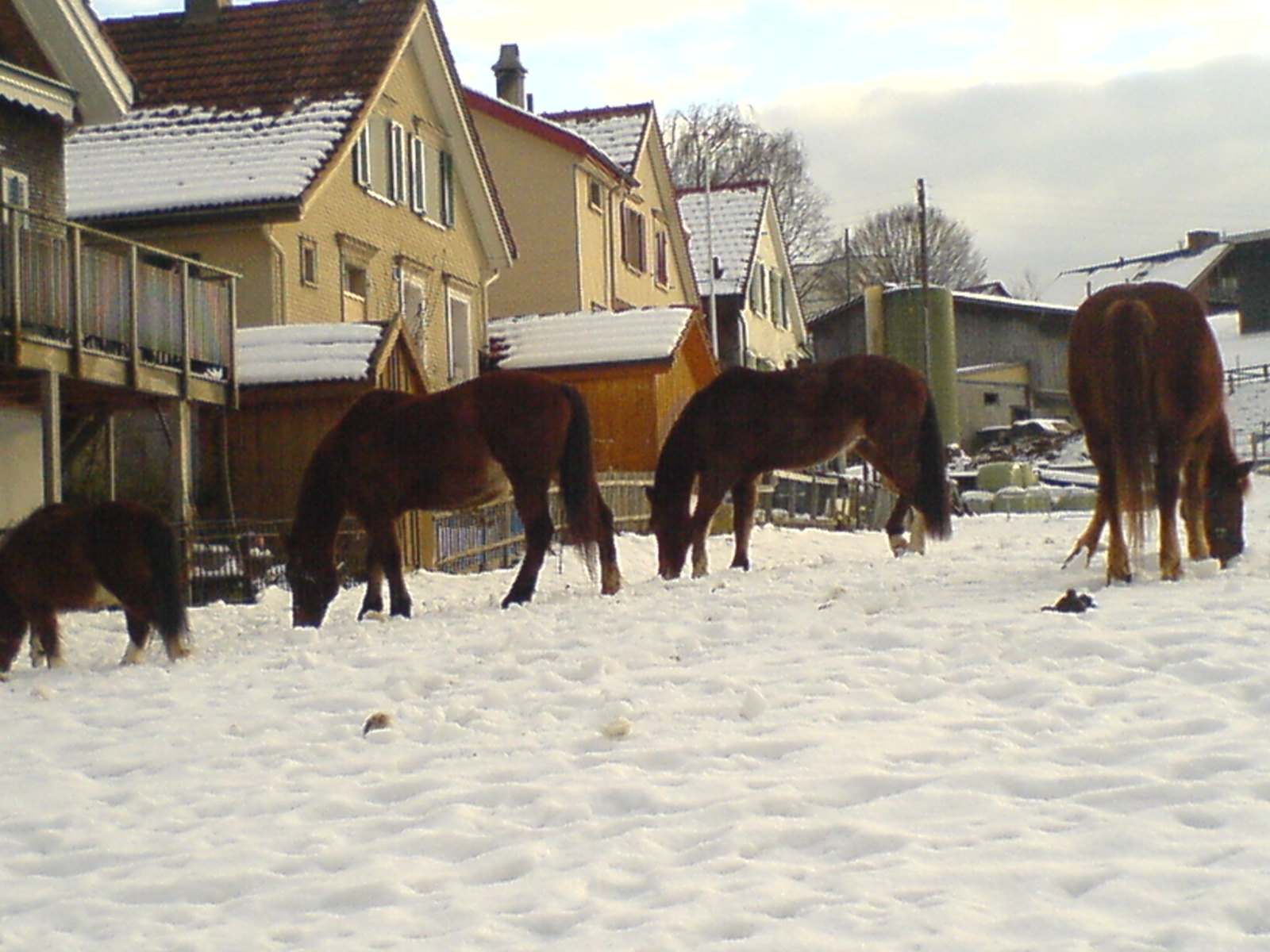This color photograph captures a serene, wintry scene featuring four chestnut brown horses, one of which appears to be a pony or colt, foraging in the snow for greenery. The horses are all positioned with their heads buried in the snow, likely searching for food, and none of them face the camera directly. Three of the horses are shown from the side, while the one on the far right is viewed from behind. The ground is a well-trampled blanket of snow, indicating the horses have been moving around the area.

In the background, a row of four two-story houses with peaked roofs stretches along the left side. These homes, mostly light beige or tan with brown shingles, display a mid-century to 1970s architectural style. Each house is accompanied by a woodshed, and there's a larger barn further to the back right, possibly accompanied by a horse trailer. A green silo or shed is noticeable in the center background, adding a touch of color to the otherwise muted winter palette.

The sky is overcast with grey clouds, though a small patch of blue sky breaks through near the top of the photo. Snow covers both the ground and the roofs of the buildings, contributing to the tranquil, chilly atmosphere. This setting is likely a ranch or a neighborhood with substantial yards, evidenced by the multiple structures and the ample snowy field where the horses roam.